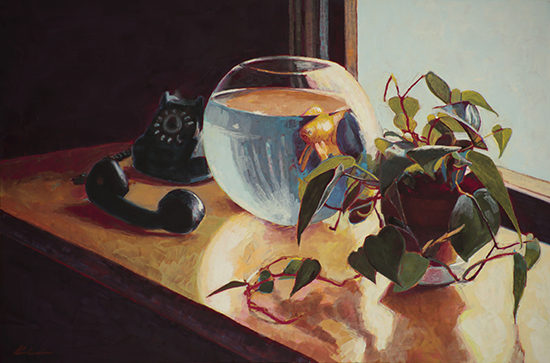This appears to be an old, likely oil-painted photograph depicting a serene still life scene on a wooden table situated in front of a frosted, bluish-gray window. Dominating the center of the table is a large, clear fishbowl containing a vibrantly bright orange goldfish, which appears somewhat oversized for the bowl. The water in the bowl is a clear blue, reflecting the goldfish's color at the surface. To the left of the fishbowl, there is a vintage black rotary telephone with the handset off the hook, placed in front of the telephone's base. On the right side, a brown ceramic pot with a white saucer underneath holds a leafy green plant with reddish branches. The plant's tendrils spill over the pot, some trailing onto the table while others stand upright. The background of the scene is quite dark, obscuring any details beyond the window's frosted glass. The overall composition, with its interplay of light and shadow, adds a timeless, almost nostalgic charm to the image.